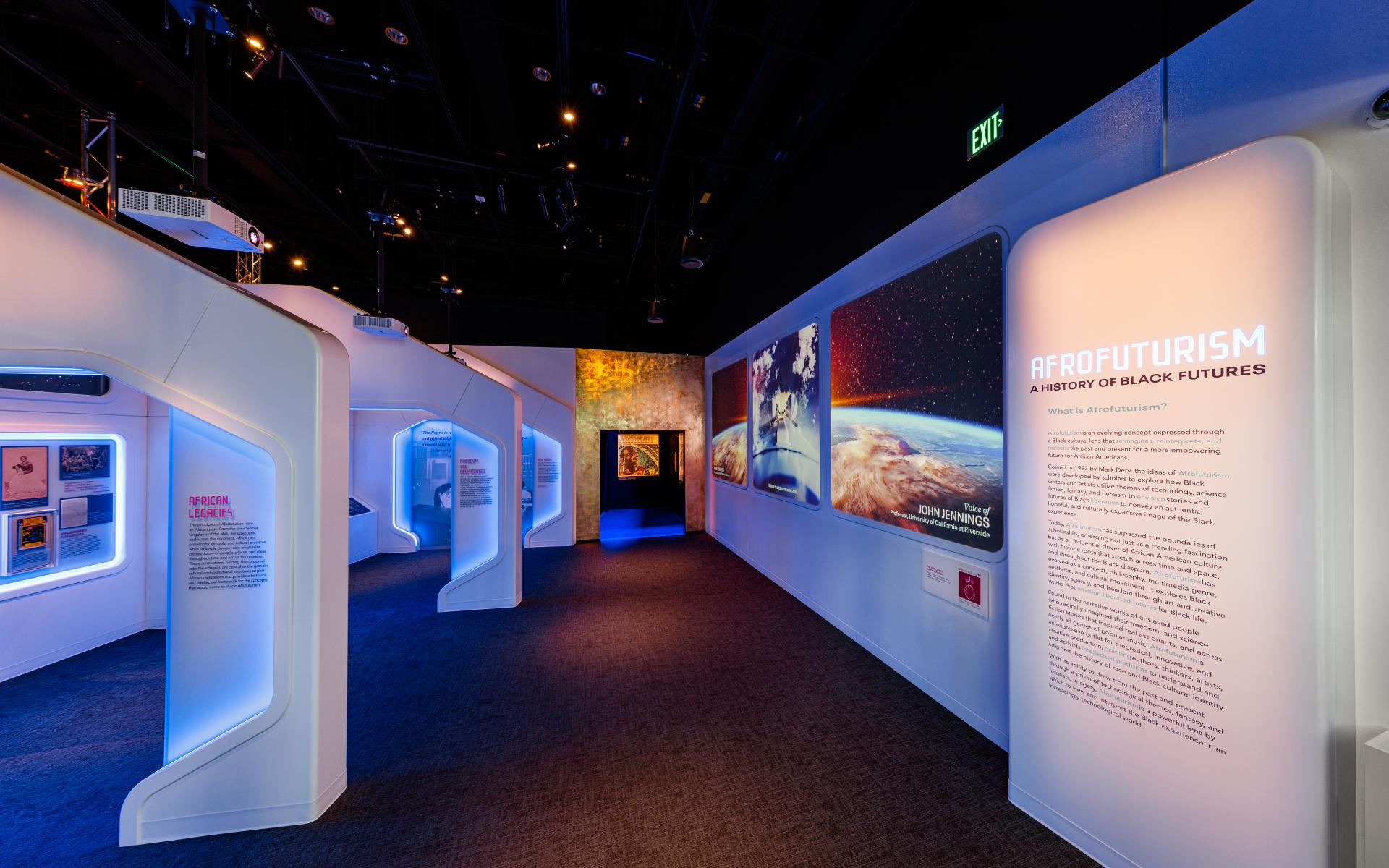The image depicts a room in a museum dedicated to Afrofuturism, a history of Black futures, as indicated by a prominently lit beige wall on the right with white and dark brown text. The wall features a few paragraphs of descriptive text under the headline "Afrofuturism" accompanied by a picture of Earth with rocks, set within a futuristic design schema. The room's ceiling is black, adorned with numerous lights that may either represent stars or serve as functional illumination, contributing to an otherworldly atmosphere.

The walls of the room are primarily white but are accentuated by purple and blue RGB lighting that adds a modern aesthetic. The museum features various exhibits, each individually lit and framed by white borders, creating discrete learning areas. Towards the back, there's a doorway highlighted with gold paint at the top, leading into interconnected rooms that also display purple and blue lighting. High above, a projector can be seen, possibly responsible for projecting images onto screens or controlling the ambient lighting.

Additionally, neon signs are present, including an "Exit" sign visible above one of the exhibits. Overall, the room combines elements of traditional museum displays with advanced, futuristic lighting and design to create an immersive experience.